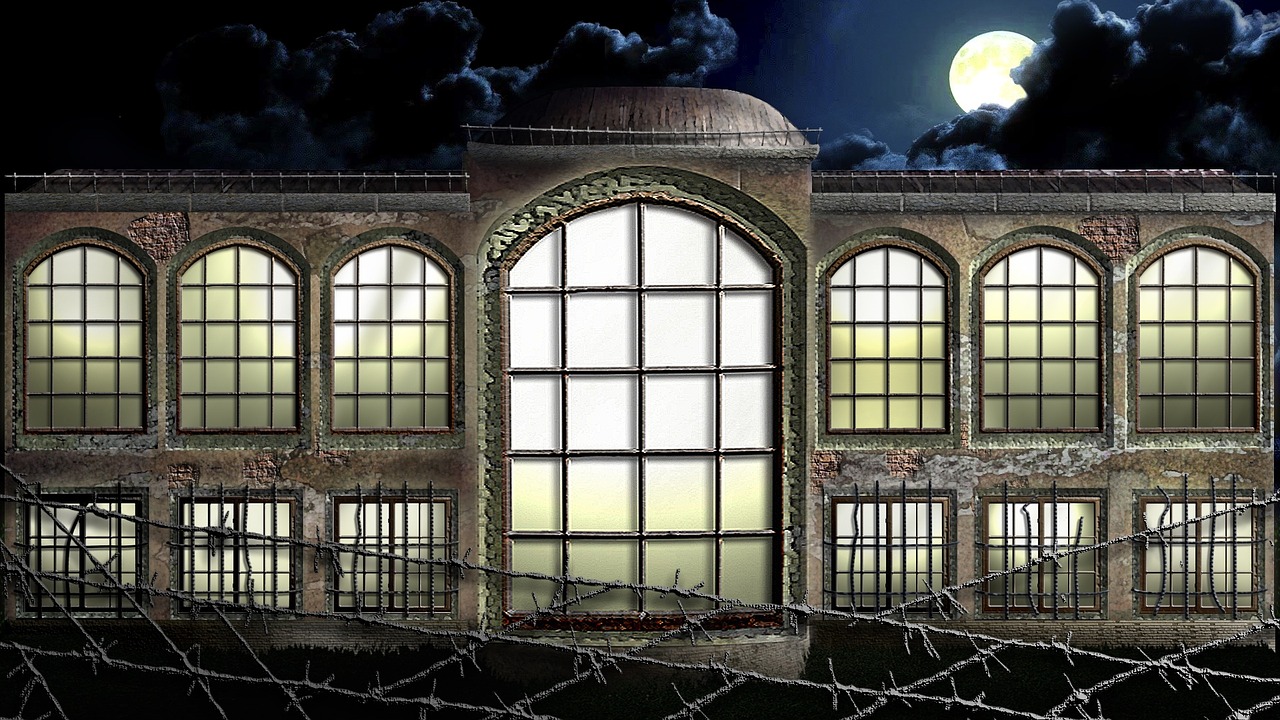The image depicts a dark and foreboding building that appears to be in disrepair. The structure is primarily made of brick and dark concrete, with parts of the facade crumbling to reveal the bricks beneath. It stands at least two stories tall, featuring large windows. The ground floor windows are square with bars across them, while the upper-floor windows are more rectangular with curved, arch-like tops. The center of the building showcases a grand, arched window that spans from the base to the top of the second floor. Crowning the edifice is a concrete dome. The night sky above is filled with ominous, almost black clouds, except for a small clear area around the moon, which is peeking through on the top right and appears orangish-yellow. Adding to the eerie atmosphere, a barbed wire fence runs along the bottom of the image, enhancing the impression of the building potentially being a prison or asylum. The windows emit a faint yellow glow, suggesting lights are on inside.